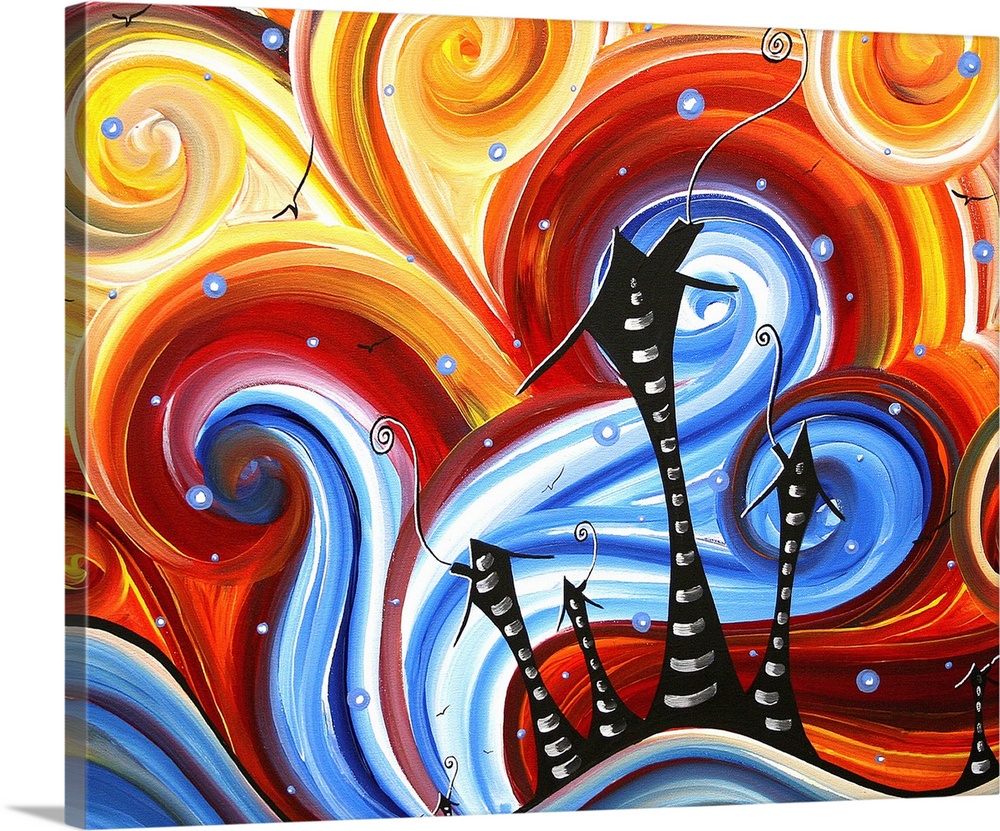This is an image of a vivid, whimsical painting on an unframed canvas, evocative of the art produced in sip and paint workshops. At the center of the composition are five intricately detailed, black and white structures, reminiscent of the fantastical styles seen in movies like Edward Scissorhands or The Nightmare Before Christmas. These towers, characterized by their skinny forms, white vertical stripes, and curlicue rooftops, vary in height with one tall tower, three of medium height, and one short one. The smallest structure is slightly off to the right. Each tower is topped with a distinctive pointed roof, some adorned with antenna-like tips and whimsical black smoke curls.

The background explodes with exuberant swirls of color, featuring sets of concentric circles in alternating hues of deep blue, vibrant yellow, passionate red, and sunny orange. These dynamic color swirls are accentuated by myriad shades within each color set, contributing to the painting’s energetic flow. The swirls sweep across the canvas, starting with warm reds, yellows, and oranges towards the top and transitioning into a palette dominated by cooler blues at the bottom. Interspersed throughout the painting are small blue bubbles with subtle white highlights, adding depth and texture to this striking abstract scene. This captivating backdrop contrasts sharply with the stark, quirky towers, combining to create a modern, fantastical landscape.